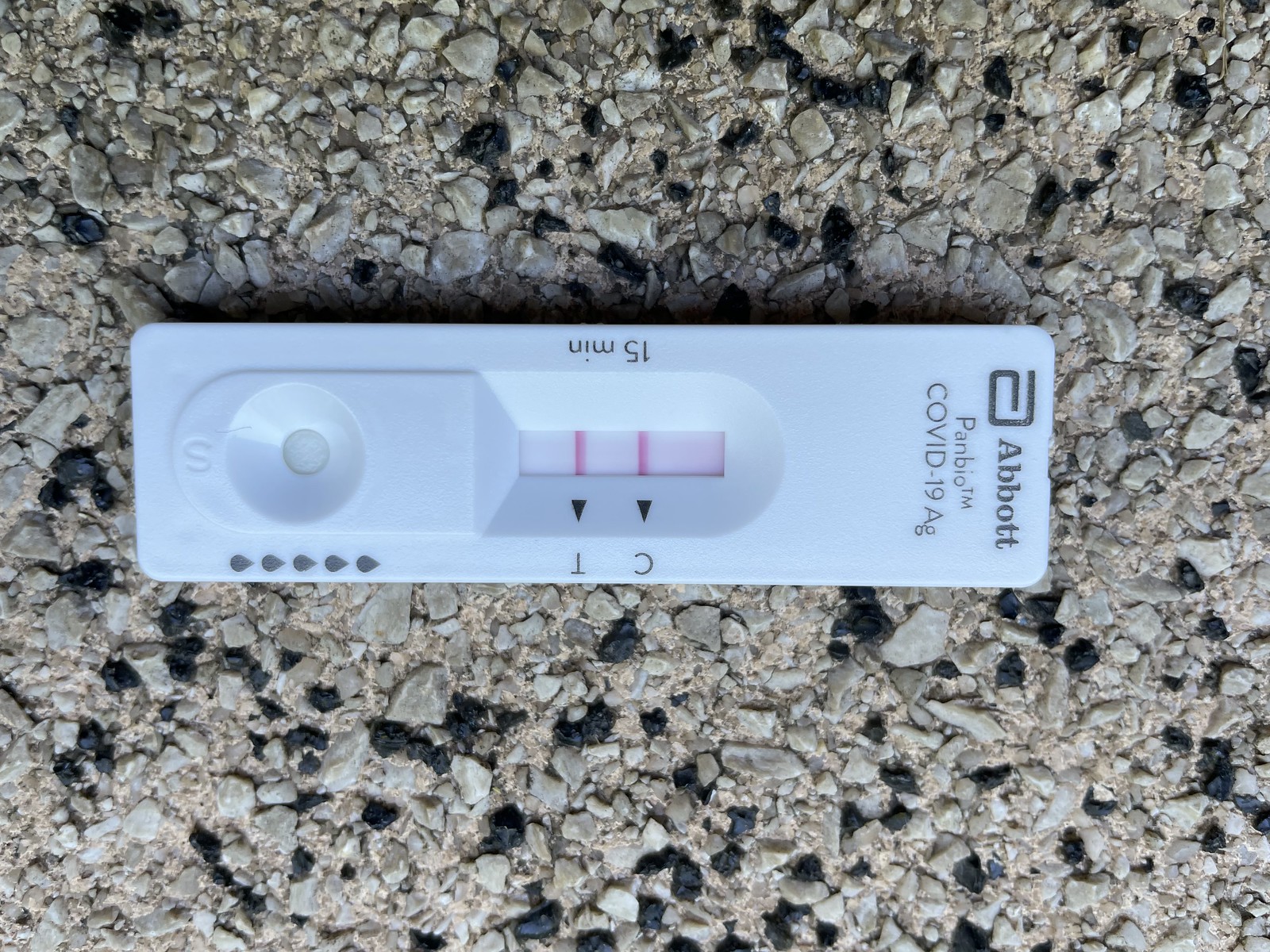This image features a countertop composed of various pebbles and stones, predominantly in shades of gray, tan, and black. Atop this countertop lies a single COVID-19 test. The test is a long, white rectangle branded with the Abbott logo. It carries the label "Panbio™ COVID-19 AG," with "AG" standing for antigen.

The test strip displays a control line (C) and a test line (T), both of which are prominent, indicating a positive result. Below the test line, there are arrows pointing to a small section marked with an "S" that contains a small indentation designed to hold a sponge-like material for absorbing liquid. This is the area where test drops are applied.

To the right, there are indicators showing that five drops are required for the test. Instructions stating "15 MIN" are printed on the opposite side of the rectangle, signifying that the result should be read after 15 minutes. Both the control and test lines are pink, verifying a positive result for COVID-19.